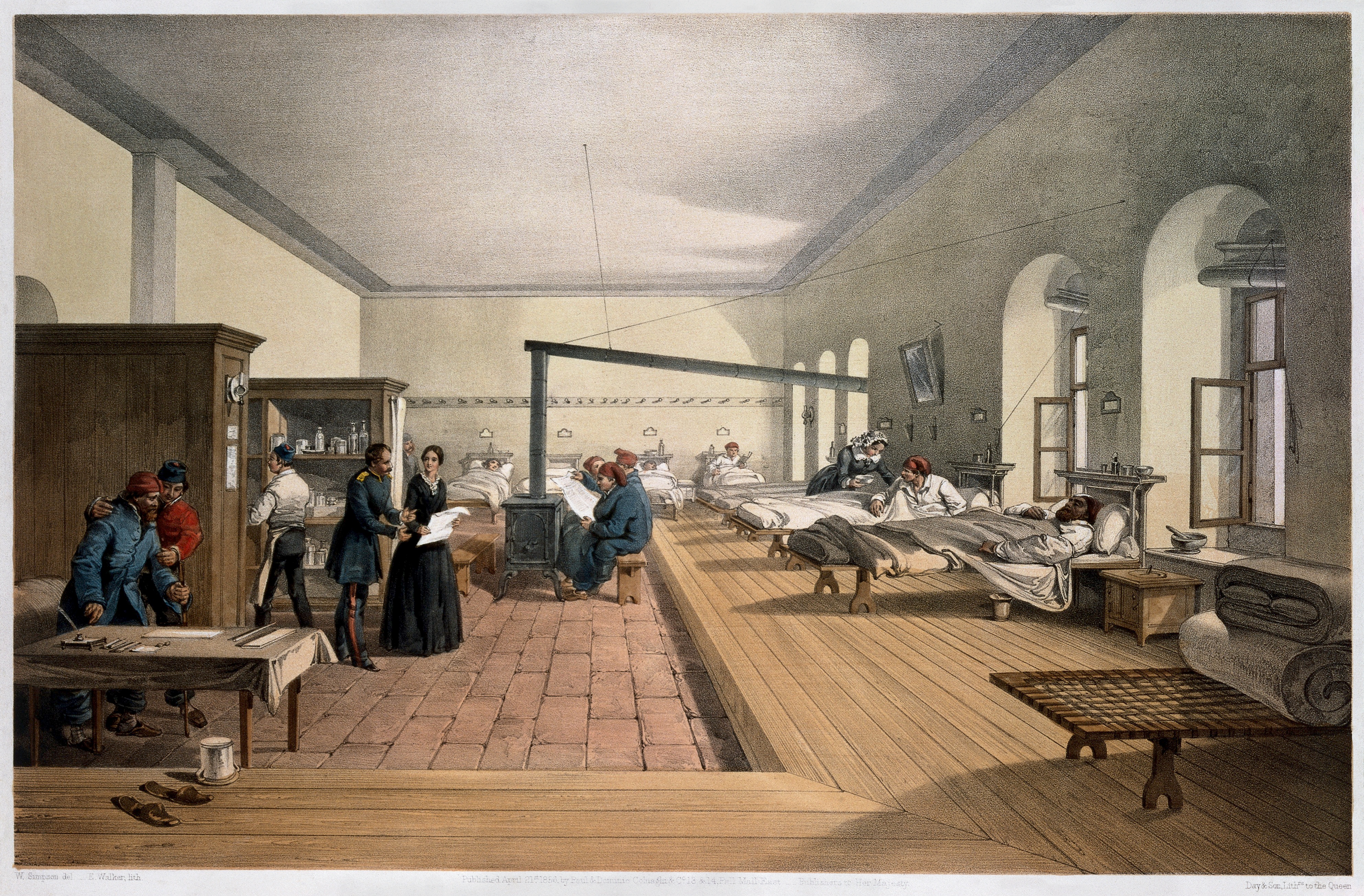This meticulously detailed painting, set in the 1800s, likely during the Civil War era, depicts an infirmary inside a rectangular room that extends horizontally. A thin gray border encases the entire scene, with inscriptions at the bottom left reading "W. Simpton Walker T.I.T.H" and at the bottom right "Day D. San Tithe to the Queen." The room is adorned with light yellow walls and features a combination of pale red brick and brown wood flooring. 

Along the right side, open windows with arched tops are set into deep brown frames, their white curtains pulled up, allowing light to stream onto a series of old-style rope cots. Some of these beds are occupied by patients, their heads resting on pillows, while the bedding is either rolled up mattresses and blankets or occupied by people. 

In the center of the room stands a large gray heating stove. At the foreground of the right side, a Union soldier in blue uniform converses with a nurse in a long black dress; both are holding white papers. Tall shelving cabinets with various jars line the room, contributing to the medical atmosphere. To the left, a woman in red tends to an injured man, also in a blue coat, near a table cluttered with writing instruments and papers. The interplay of the detailed elements captures the essence of a bustling, historical military hospital.